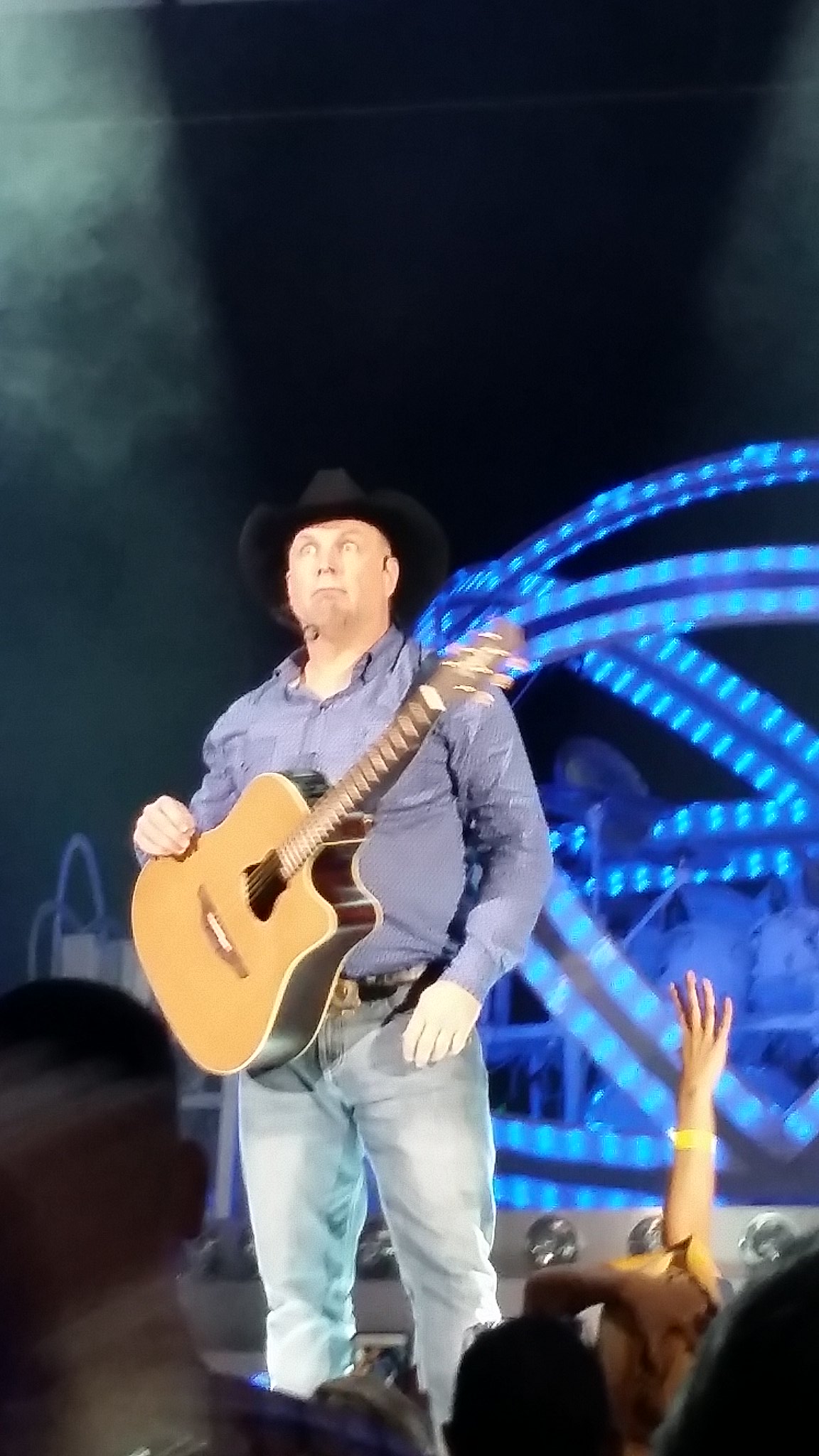In this dynamic image, country music icon Garth Brooks is captured mid-performance on stage. Dressed in a long-sleeved lavender or blue shirt, light-colored jeans, a black cowboy hat, and a gold belt buckle, he stands with an acoustic guitar slung over his shoulder. Garth's wide-eyed, surprised expression suggests he's reacting to something in the audience or the environment around him. The scene is framed from the perspective of an audience member, with a woman raising her hand adorned with a yellow bracelet and a man partially blocking the view in the foreground.

The stage is set with an intricate circular structure behind Garth, adorned with blue LED lights that create a mesmerizing backdrop. This blue structure resembles a globe and is vividly illuminated, drawing attention. Additional elements in the background include what seems to be a silver platform with unlit lights and the top of another person's head, hinting at a larger, bustling setting. The environment appears to be a blend of indoor and outdoor elements—possibly an open-air arena—with dark skies and clouds visible above, and smoke illuminated by a spotlight adding to the atmospheric setting.